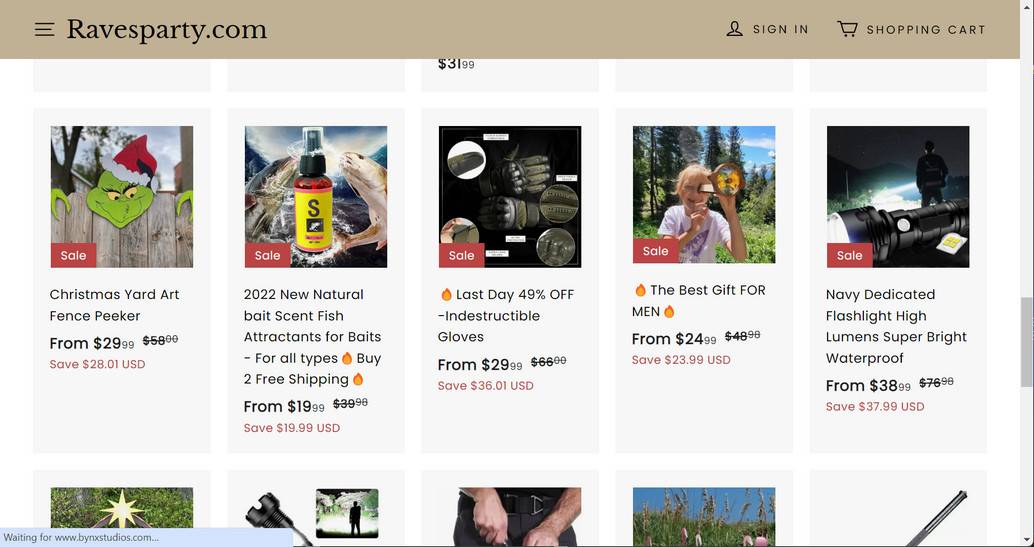Screenshot Description:

This image captures a screenshot of the e-commerce website ravesparty.com. The header of the website features a beige background. Positioned on the left side of the header is the site’s name, "ravesparty.com", written in a sleek black font. Adjacent to it on the left are three horizontal black lines, indicating a drop-down menu. On the right side of the header, there are icons and text for "Sign In" and the shopping cart.

Below the header, the background transitions to white, displaying a selection of products typical of novelty gift items. There are five product images in the main viewing area:

1. **Christmas Yard Art Fence Peeker**: Depicts an image resembling the Grinch from Dr. Seuss’s classic, designed to hang over a fence.
   
2. **2022 New Natural Bait Scent Fish Attractants for Baits**: Shows a small bottle with a yellow label, presumably containing fish attractant scent.
   
3. **Indestructible Gloves**: Features a pair of dark gray gloves set against a black background, marketed for their durability.
   
4. **Best Gift for Men**: Though the title suggests an ideal men's gift, the product is obscured, showing only an ambiguous image of someone looking through a large lens.
   
5. **Navy Dedicated Flashlight, High Lumens, Super Bright**: Provides a side view of a sleek black flashlight, indicating its powerful brightness.

The bottom part of the screenshot hints at another row of product images, with only the top edges of these items visible, suggesting there is more to explore on the webpage.